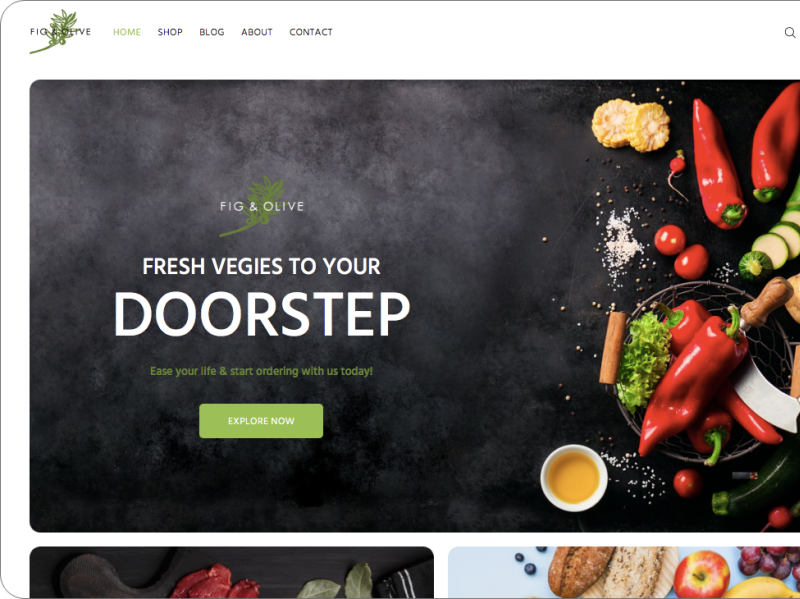The image showcases a partial view of the Fig and Olive website, focusing primarily on the left-hand side of the webpage. In the upper left corner, the Fig and Olive logo is prominently displayed, featuring the brand name overlaying a delicate olive branch, all rendered in green tones. Adjacent to the logo, a navigation menu is highlighted, with the "Home" tab illuminated in light green, followed by links to "Shop," "Blog," "About," "Connect," and "Contact." To the far right of the menu, a search icon in the shape of a magnifying glass is present.

Beneath the navigation bar, a large central media banner displays another iteration of the Fig and Olive logo on the left, accompanied by the tagline "Refresh veggies to your doorstep," though "veggies" is incorrectly spelled as "begies." Below this slogan, the phrase "Ease your life and start ordering with us today" invites users to take action, featuring two prominent buttons labeled "Explore" and "Now," both highlighted in green.

The right-hand side of the image visually emphasizes fresh produce, including an assortment of serrano peppers, corn, olive oils, parsnips, sea salt, grape tomatoes, and chopped cucumbers. Along the bottom, partially visible images of food products, such as an apple, grapes, a partial banana, and some bread, hint at more offerings available on the website.